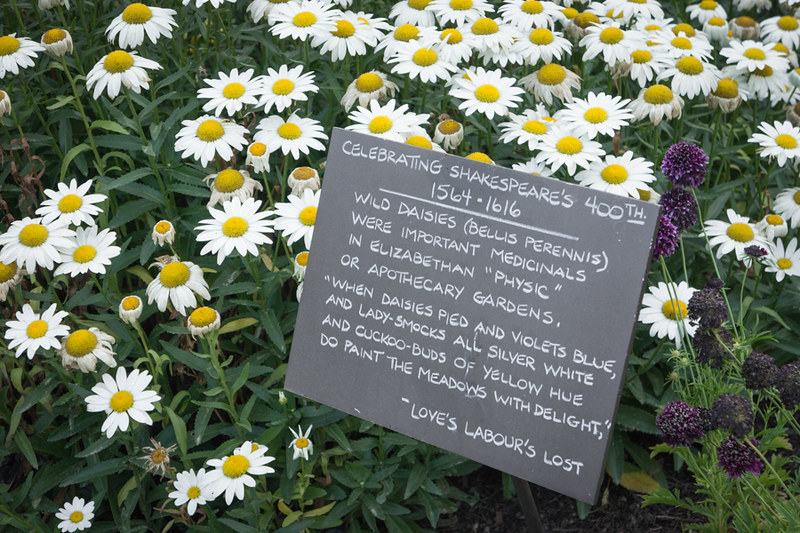The image showcases a garden filled predominantly with white daisies, each with a bright yellow center, extending throughout the scene. Interspersed among the daisies, particularly in the lower right corner, are purple weed flowers with long green stems. In the center of the image, there is a gray sign with white lettering. The sign reads: "Celebrating Shakespeare's 400th, 1564-1616. Wild daisies, Bellis perennis, were important medicinals in Elizabethan physic or apothecary gardens." Below, a line separates the main text from a quote: "When daisies pied and violets blue and lady smocks all silver white and cuckoo buds of yellow hue do paint the meadows with delight." This quote is attributed to Shakespeare's "Love's Labour's Lost." The background and surroundings of the sign emphasize the natural beauty and historical significance of the plants depicted.